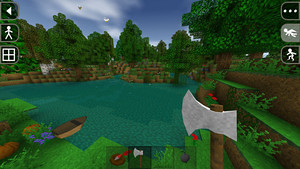A vivid Minecraft scene unfolds, depicting a natural environment composed of iconic, blocky shapes. Dominating the foreground, a character is equipped with an axe, although only the tool is visible. Adjacent to the character's implied location, a small boat rests on the ground, and tufts of pixelated grass sprout near their feet. Directly ahead lies a shimmering pool of water. In the background, rolling dirt mounds topped with verdant grass and blocky trees stretch towards a bright blue sky, specked with fluffy white clouds. Birds, one white and one black, flutter leisurely in this serene setting.

The image further immerses the viewer with a detailed user interface (UI). In the bottom section, an inventory bar displays the axe and several other item slots. The top left corner houses a mini-map or character grid, featuring a humanoid figure and directional arrow, suggesting navigational aids. On the top right, three white dots accompany a floating white character icon, another similar icon below indicating possible player actions or NPC activity, all framed by a gray square, hinting at some in-game notifications or settings.